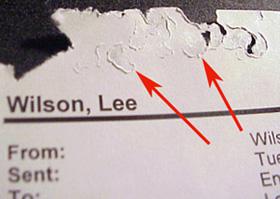This photograph showcases a piece of old, tattered paper with significant focus on its upper edge, marked by two prominent red arrows pointing towards the damage. The paper displays the name "Wilson, Lee," underlined with a straight black line, and below this, phrases like "from:", "sent:", and "to:". The background text, partially obscured, includes segments beginning with "W-I-L-S," "T-U-E," and "E-N". The damage at the top of the paper includes scattered, rounded tears that resemble incomplete hole punches, possibly giving the appearance of an animal bite. The paper lies against a black background.